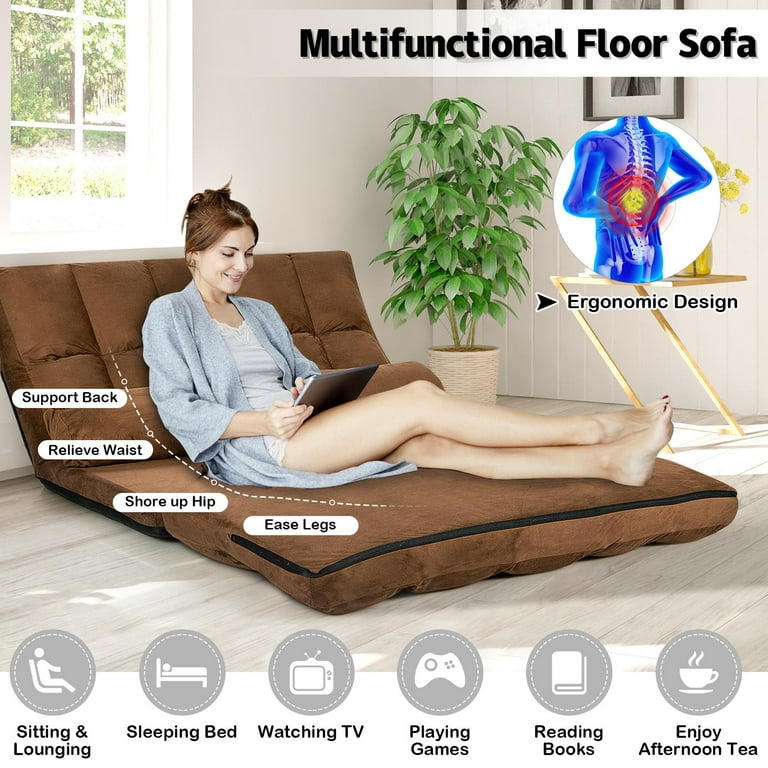In a cozy indoor setting, a white woman in her 30s is seen reclining comfortably on a Multifunctional Floor Sofa. This innovative piece of furniture, essentially a large brown cushion propped against a wall, supports her as she lounges barefoot in a blue bathrobe over a white shirt and shorts. The room, likely a living room, features a light brown potted plant in the corner and a white-framed window above her. A text overlay in bold black letters reads "Multifunctional Floor Sofa," accompanied by an ergonomic design graphic highlighting back pain relief. Ovals below the graphic list the benefits: support back, relieve waist, shore up hip, and ease legs. Additional icons detail its versatile uses, including sitting, lounging, sleeping, watching TV, playing games, reading books, and enjoying afternoon tea. The sofa’s brown cover, zipper-enabled for easy washing, emphasizes its practicality and user-friendly design.